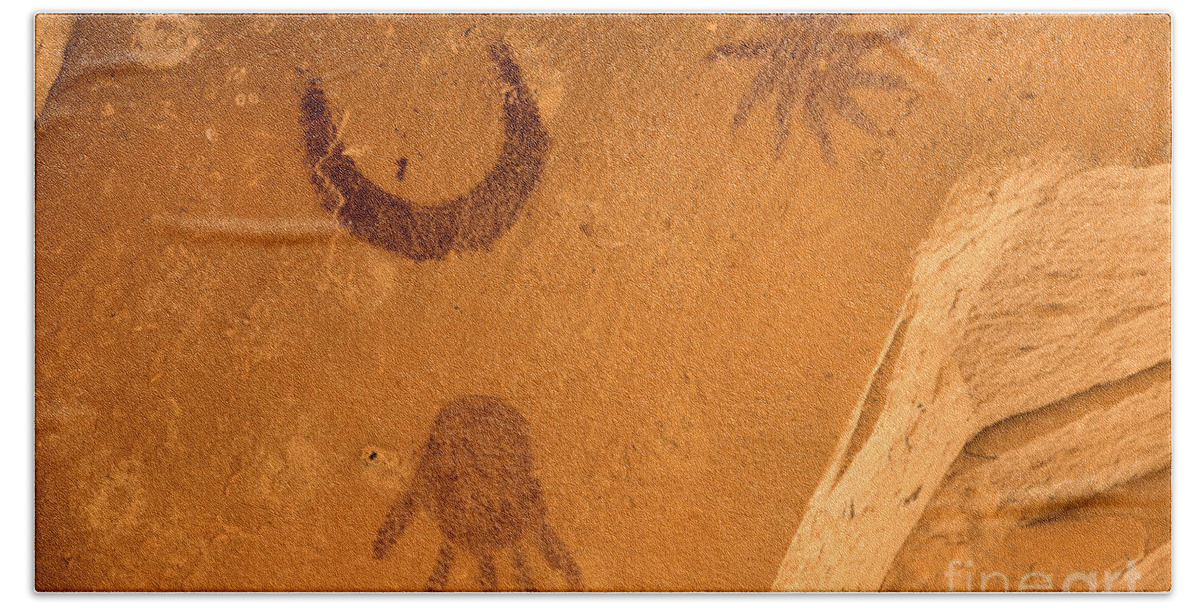This photograph captures an ancient-looking stone wall, possibly made of clay or sandstone, displaying simplistic drawings. The image is predominantly in shades of brown and features a smooth surface punctuated with varied textures, faint white diagonal lines, and a rough, protruding area on the right side in a lighter, sandy color. The wall also contains subtle contour variations with specks and cracks, adding to its aged appearance. Highlighted on this smooth surface are three striking drawings: an upside-down, uniform brown left handprint with the thumb and four fingers extending clearly; a dark brown crescent moon shape positioned slightly to the left in the top middle; and an eight-armed star-shaped symbol located in the top right of the image, though slightly cropped. In the bottom right corner, partially cut off, is a watermark reading "fine art."